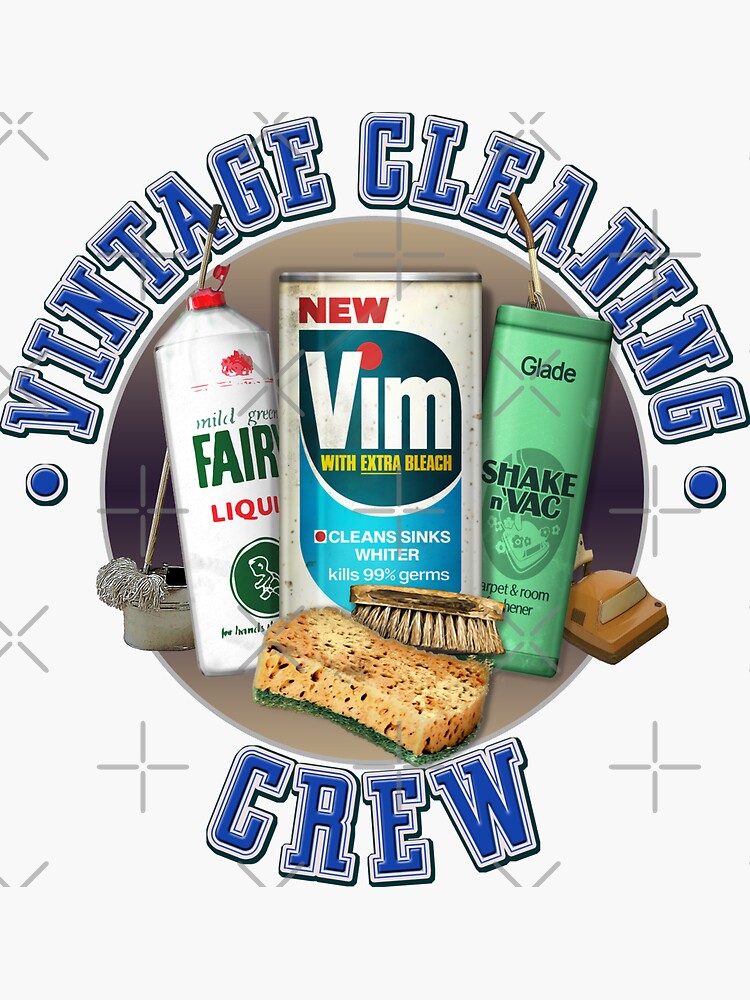The advertisement showcases a vintage cleaning crew theme with a vibrant, cartoon-style design. The top of the circular image features the text "Vintage Cleaning" in bold, curved black font, flanked by dots under the "V" and "G". At the bottom, the word "Crew" is displayed in blue text. In the center, a collection of cleaning supplies stands out against a light gray background overlaid with X and plus signs resembling watermarks. Prominently featured is a can of "New Vim with Extra Bleach," which boasts the ability to clean sinks whiter and kill 99% of germs. To the right, a green bottle of "Glade Shake and Vac" carpet and room cleaner is highlighted, while on the left, a mild green "Fairy Liquid" cleaning solution can be seen. Surrounding these products are additional cleaning essentials, including a worn yellow sponge with a green underside, a few sponges, soaps, and scrubs, all rendered in a colorful and lively cartoon style.